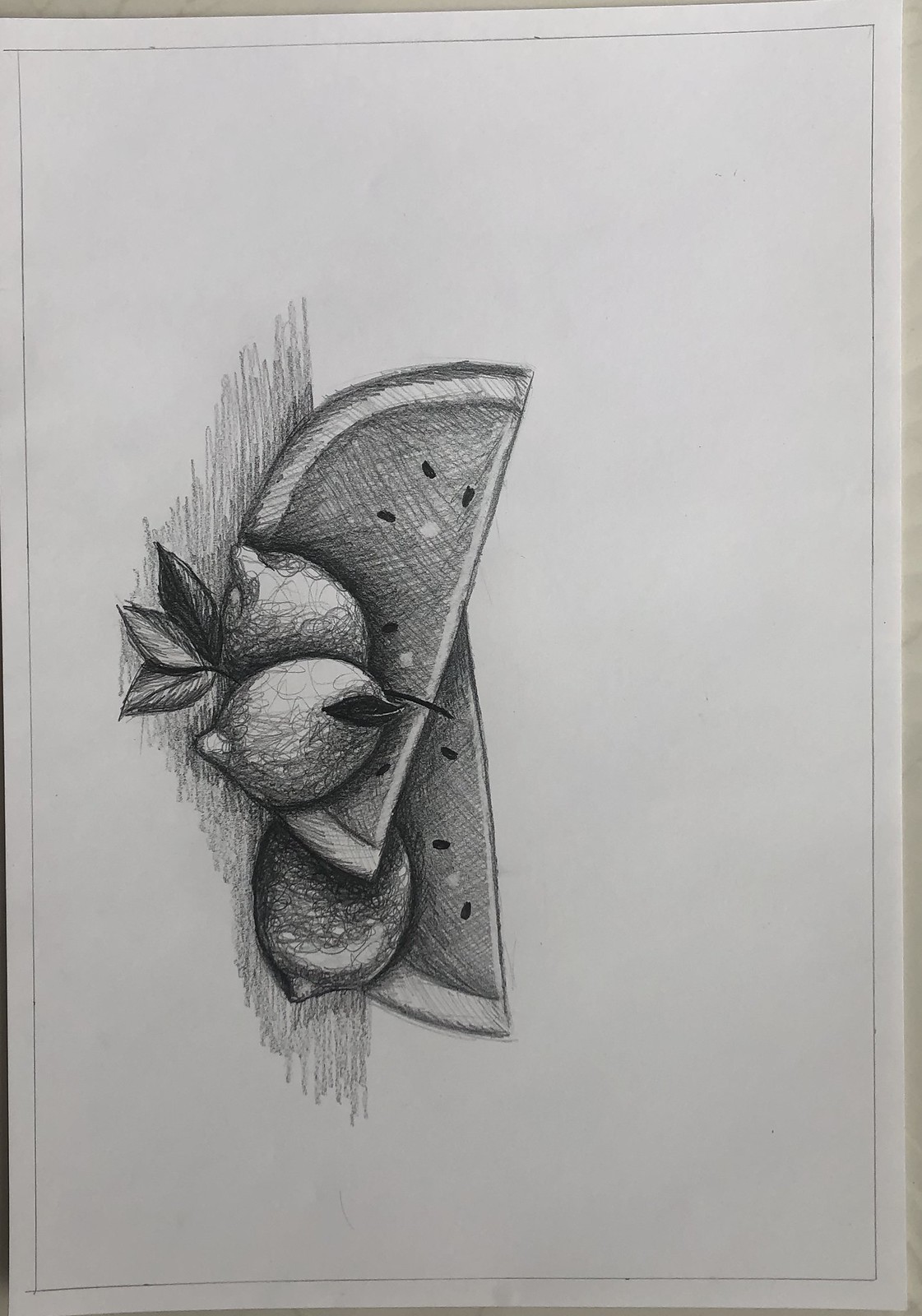This pencil drawing, originally intended to be viewed horizontally but presented here vertically, captures a carefully arranged still life of various fruits. Predominantly featuring two large slices of watermelon, the composition also includes several citrus fruits—likely lemons or limes, though the black and white medium leaves their exact identification open to interpretation. In the foreground, three leaves, possibly mint or associated with the citrus fruits, add an additional layer of texture to the arrangement. The artist employs meticulous shading and cross-hatching techniques to add depth and realism, enhancing the three-dimensional quality of the fruits and leaves. The interplay of light and shadow highlights the precision and artistry of the pencil work, inviting viewers to appreciate the intricate details and thoughtful composition.